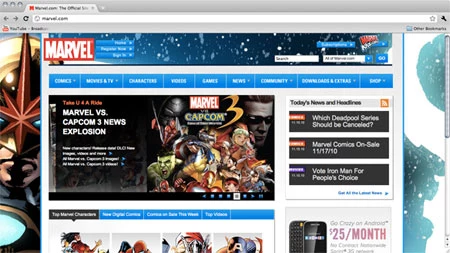The image displays various elements related to Marvel and Capcom, with a prominent superhero theme. On the left side, there is a detailed depiction of a superhero featuring a star emblem on his head, blue eyes, a gold mask at the top, and a blue chest armor. The central part of the image showcases a group of superheroes, although most are blurry except for one on the right who is wearing sunglasses. A possible Hulk figure is discernible on the left with a green hue.

The right side of the image includes a blue leaf pattern with a white swirl and a visible scroll bar. At the top, there is a browser's address bar indicating only one tab is open. Various texts are also scattered across the image: "Marvel," "Marvel Capcom," "Marvel vs. Capcom 3," "News Explosion," "Which Develop Pool Series Should Be Cancelled," "Marvel Comics On Sale 11-17-2010," and "Vote Iron Man For People's Choice $25 A Month," though some parts remain too blurry to read.